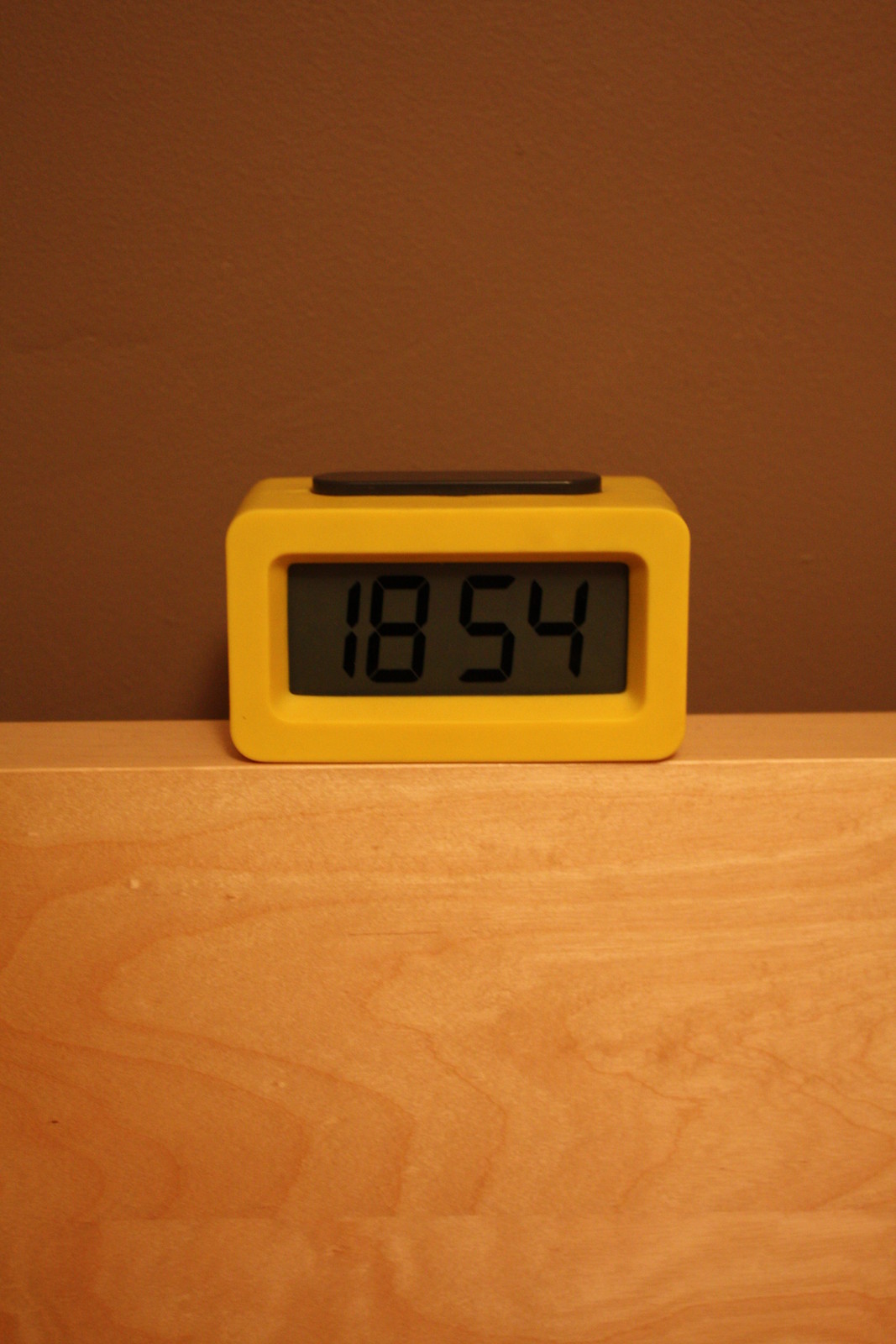The focal point of the image is a large digital alarm clock displaying the time "1854," indicating 6:54 p.m. in military time. The clock's digits are prominently displayed in black against a slightly lighter dark black background. The clock has an exterior casing that appears to be white, possibly yellowed due to the lighting, or it might inherently be a yellow shade. A black button, likely a snooze button, is situated on the top of the clock. The clock is positioned on a varnished wooden ledge, which is adjacent to a wall. The wood has a notable thickness, almost matching the depth of the clock, and shows both its top edge and vertical face. The wall behind the ledge is painted in varying shades of brown, ranging from light to dark brown, influenced by the lighting in the scene.